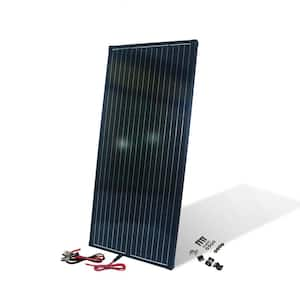This image depicts a black rectangular panel, which appears to be a solar panel. The panel stands vertically, slightly tilted to the right, and features vertical white stripes running along its surface. It has a white border framing it. At the bottom of the panel, a cord can be seen emerging, starting as black and transitioning to red. To the left, there are additional wires or possibly alligator clips in various colors.

The background of the image includes scattered screws, bolts, and other small machinery components. The panel reflects two distinct white dots of light, suggesting a light source illuminating it. The panel casts a shadow on the white surface behind it. The photograph seems to be low in resolution, which makes the finer details of the objects challenging to discern.